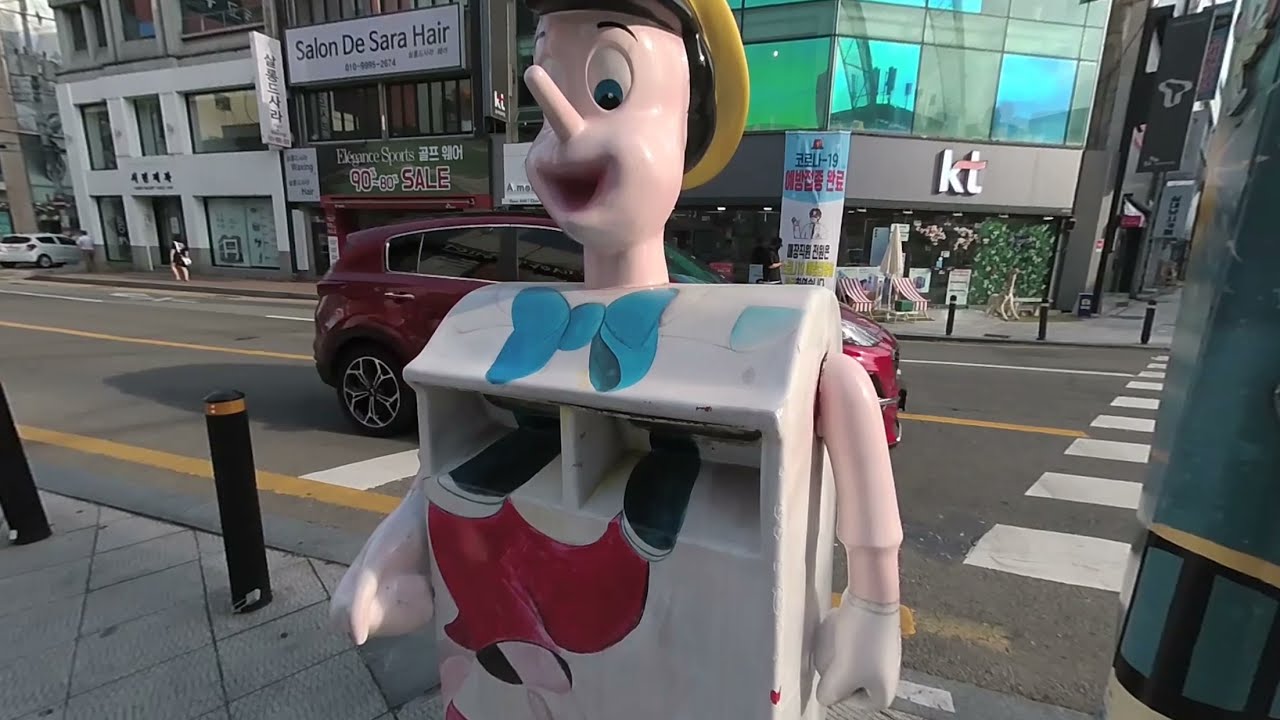In the foreground, there is a striking statue resembling a large, black garbage can or a mailbox, painted to look like Pinocchio. This unusual statue features a white, square body adorned with a blue bow tie, red accents at the bottom, and protruding arms, topped with the unmistakable Pinocchio head complete with a long nose. The setting appears to be a busy multi-lane street in the middle of a city, seen from the perspective of a sidewalk near a crosswalk. Surrounding the statue, there are concrete blocks forming a walkway that leads to the street where several cars are visible, including one directly behind the statue. The background showcases various buildings and shops, one of which has "KT" labeled above its doors and another with a sign that reads "Salon de Sarah Hare." Many of the signs feature foreign writing, suggesting an Asian influence, possibly Korean, hinted by the abundance of Asian symbols. The scene is set outdoors in daylight, with noticeable colors including gray, black, white, red, and blue among others.